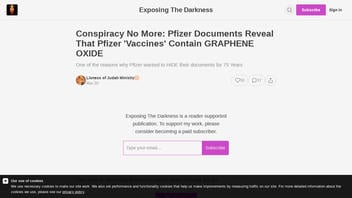**Caption:**

The image features a webpage with a predominantly white background and black text. At the top, large black text reads, "Exploring the Darkness." In the top right corner, a purple button with indiscernible text is positioned next to a magnifying glass icon. On the left-hand corner, there's a small logo resembling a fire, contained within a black box with a red element.

Below the main heading, a secondary heading states, "Conspiracy: No More Pfizer Documents Reveal that Pfizer Vaccines Contain Graphene Oxide." The page appears to begin an article, but the text is too small to read clearly. 

Towards the bottom of the page, there's a white text input box accompanied by a purple button, potentially for user interactions. At the very bottom, a black bar spans the width of the page, containing some white text that is also too small to discern.

The overall layout contrasts the white background with black and purple elements, drawing attention to the text and interactive features.